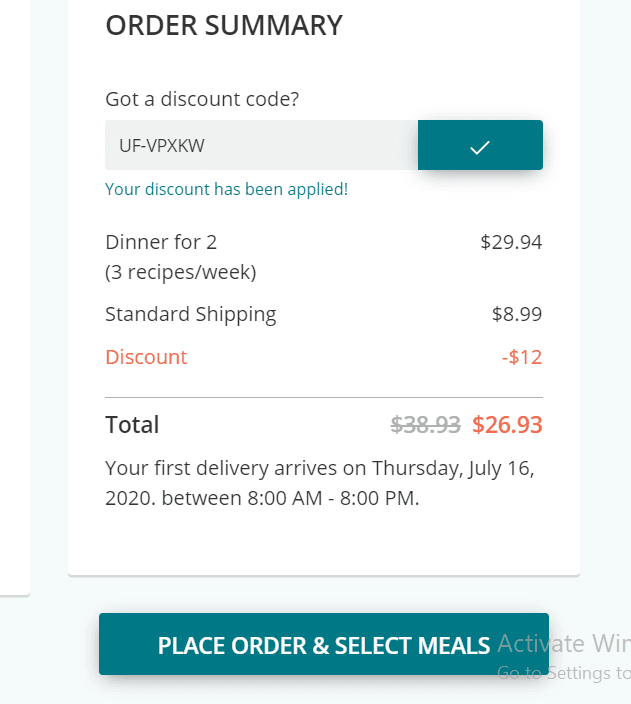At the top of the image, **Order Summary** is prominently displayed in bold black letters. Approximately two inches below, on the left side, there is a section labeled "Discount Code?" alongside a long gray rectangle containing the text **UF-VPXKW**. To the right of this rectangle, there is a green box with a white check mark, followed by the text **Your discount has been applied!** in green.

Below this section, about an inch or two down, there is an itemized list showing **Dinner for Two** priced at **$29.94**. To the right of this, it notes **3 recipes/week, standard shipping**. Further down, the word **Discount** appears in red, with a negative sign and **-$12.00** in red text to the right.

A long horizontal line separates the items listed above from the total amounts. The initial total, **$38.93**, is marked through in red. Below it, the adjusted total **$26.93** is displayed in bold red. Additional text states, **Your first delivery arrives on Thursday, July 16th, 2020, between 8 a.m. and 8 p.m.**

Finally, approximately three to four inches down from the total, a long green rectangle spans the width of the image. Inside this rectangle, bold white text reads: **Place Order and Select Meals**.